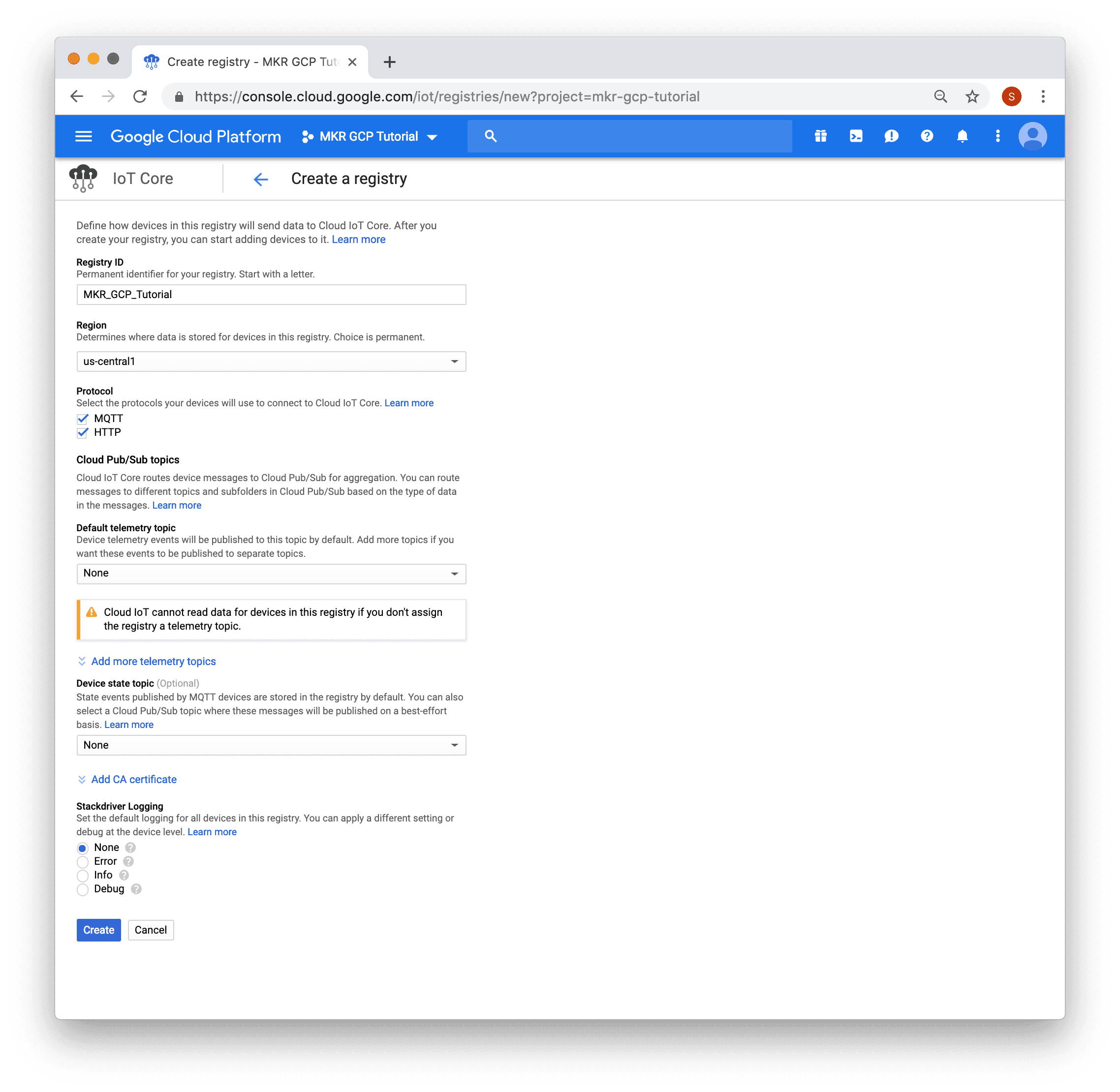The image depicts a screenshot of a Google Cloud Platform web console page, specifically within the "MKR GCP Tutorial" project. At the top, the browser tab features an icon of rainy clouds and a truncated title: "Create Registry MKR GCP TU." The header in the blue rectangle prominently displays "Google Cloud Platform," followed by the project name "MKR GCP Tutorial." Below this, a black cloud icon is visible alongside the text "IOT Core."

On the left side, the console's sidebar can be seen, featuring different navigation options. The primary section in view is titled "Create a Registry," which appears in bold black text with a left-pointing arrow beside it.

The main content area on the right is partially blank, particularly towards the bottom. However, there are several form fields and options listed, including "Registry ID," "Region," "Protocol," "Cloud Pub/Sub topics," and "Default telemetry topic." Notably, a warning message states, "Cloud IOT cannot read data for devices in this registry if you don't assign the registry a telemetry topic." The user has selected "None" for one of the options, and there is a visible button labeled "Create" likely intended to finalize the registry creation process.